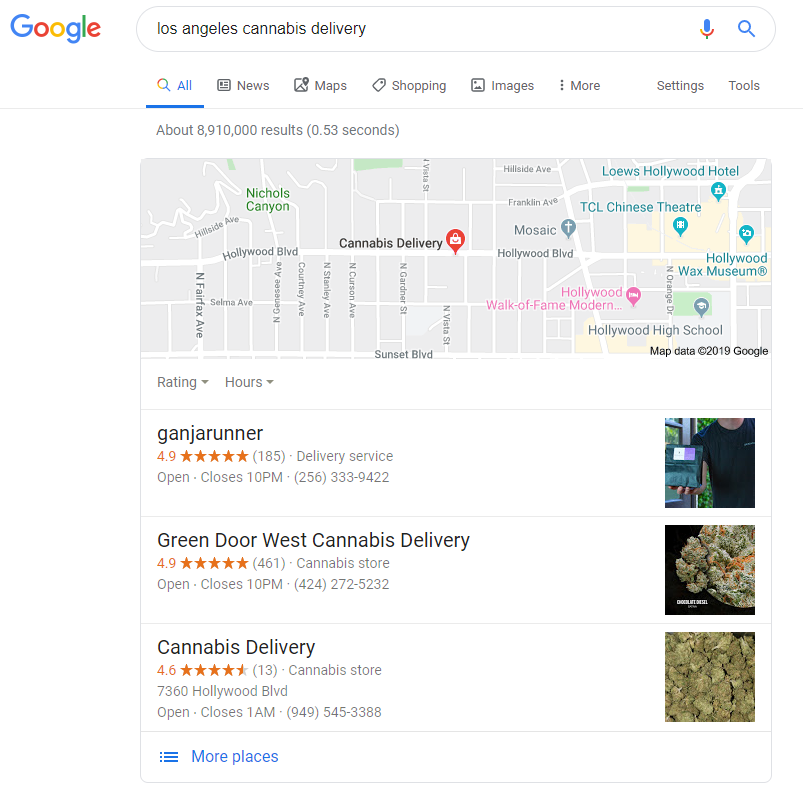A detailed screenshot of a Google search query for "Los Angeles Cannabis Delivery" is displayed against a completely white background. In the top left corner, the colorful Google logo is clearly visible, followed by the search box containing the typed query in black text, accompanied by a microphone icon and a blue search icon. Below the search bar, the standard Google menu is displayed with "All" selected in blue. Adjacent menu options include News, Maps, Shopping, Images, More, Settings, and Tools. The search yields approximately 8,910,000 results in 0.53 seconds. 

Beneath this, there is a rectangular map showcasing a red icon labeled "Cannabis Delivery" centrally positioned, with various local stores and streets also marked. Below the map, a white bar features two dropdown menus labeled "Rating" and "Hours." The search results list three cannabis shop options:

1. **Ganja Runner**: A delivery service rated 4.9 stars. To the right, there's an icon depicting a person standing inside a shop.
2. **Green Door West Cannabis Delivery**: A cannabis store also rated 4.9 stars. An image of cannabis is shown on the right.
3. **Cannabis Delivery**: A cannabis store with a 4.6-star rating, illustrated with a picture displaying numerous pieces of cannabis.

Underneath the last entry, there is a blue text link labeled "More places" accompanied by an icon with three horizontal lines indicating additional options.